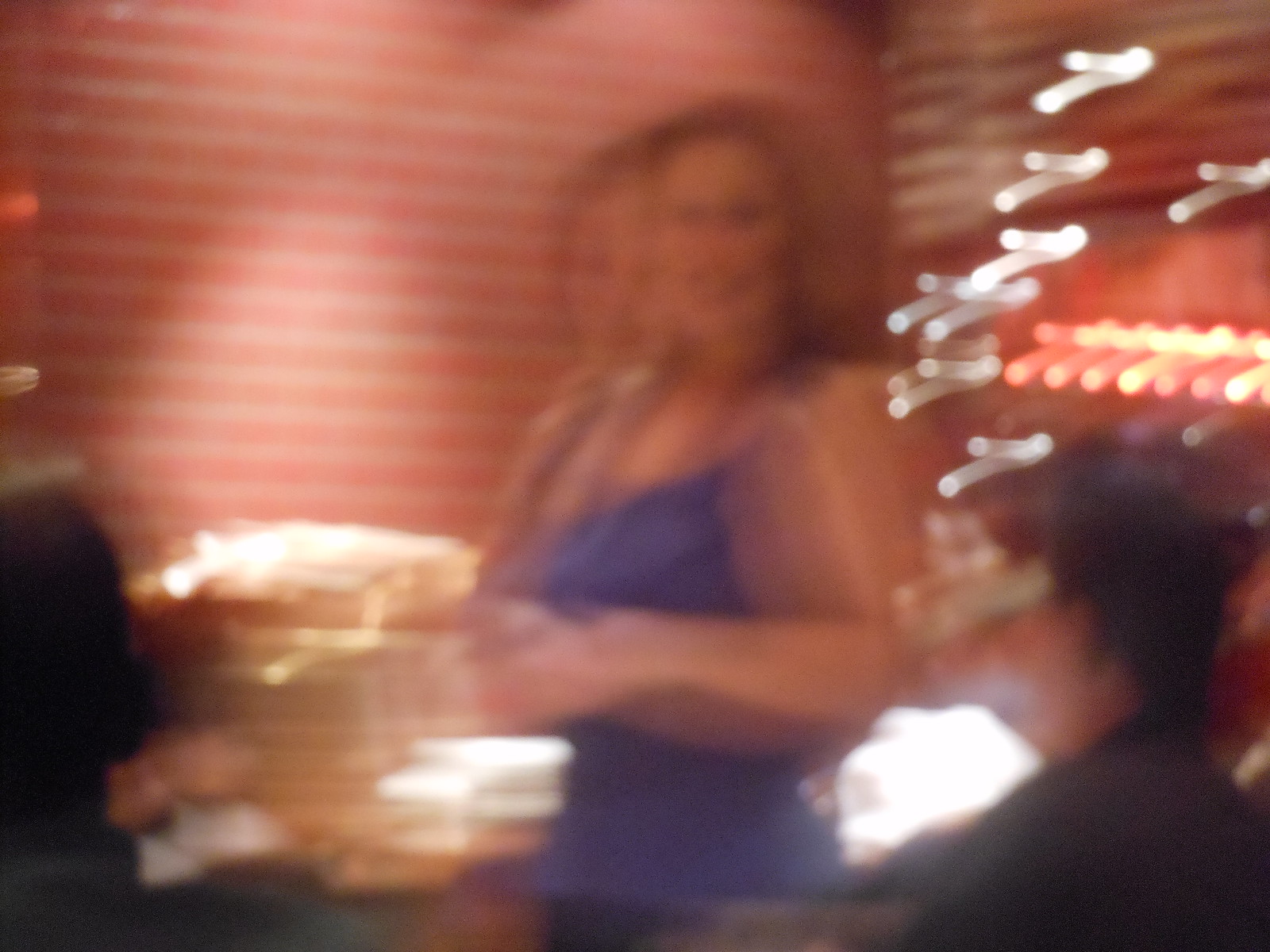This highly blurry, out-of-focus photo, possibly taken inside a restaurant, captures a dynamic scene bathed in distorted lighting. Dominating the image is a smiling woman with blonde hair, wearing a blue cocktail dress with spaghetti straps. She appears to be serving drinks or holding a tray with brightly shining glasses, though the severe blur makes the items and her movements appear doubled. Her eyes and lips are dark against her light complexion. The background features red, horizontally striped walls over a beige backdrop, likely illuminated by strip lighting and spotlights creating a vivid but unclear effect.

In the bottom right-hand side, a person with black hair in a black top is partially visible, seated, while the bottom left showcases the silhouette of another seated individual, whose hair and facial features are indiscernible. The overall scene is awash in red lines against a white background, contributing to the chaotic yet interesting visual composition.